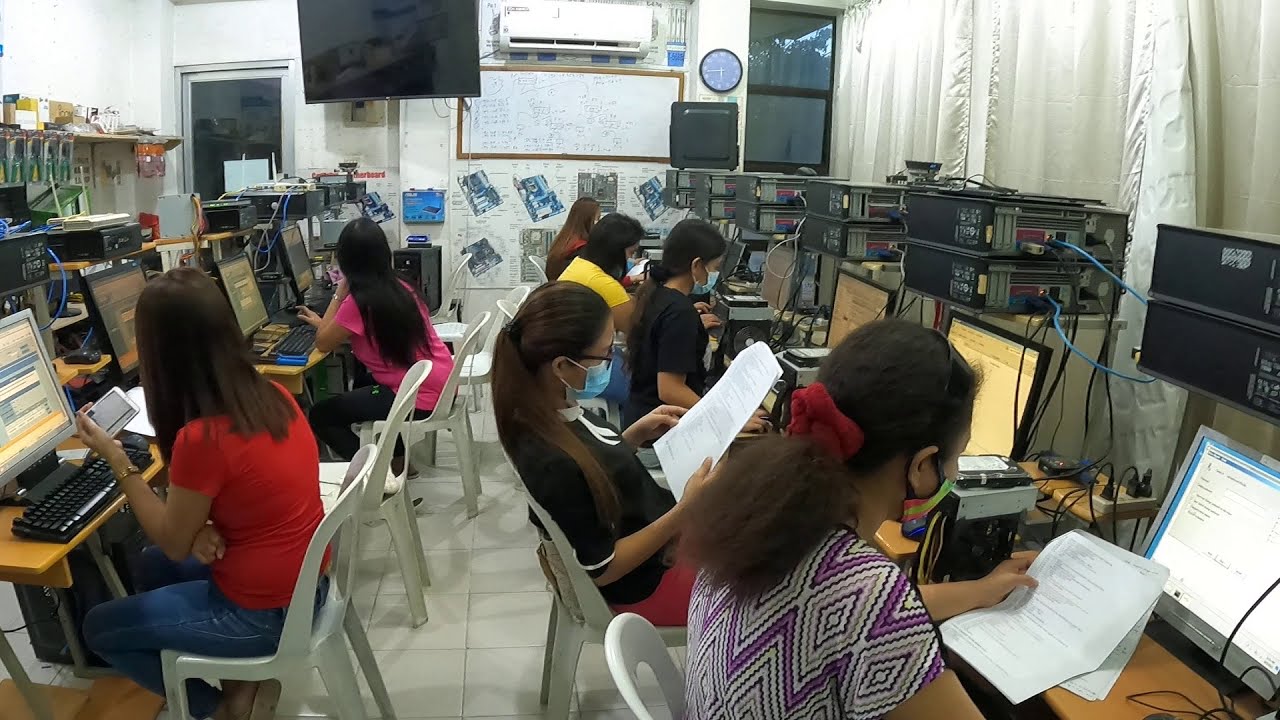The image depicts an interior view of a computer lab or office space, occupied by seven women. Each woman is seated in a plastic lawn chair at individual computer stations, arranged in two rows along the left and right sides of the room. Each station is equipped with dual desktop computers and a lower desk monitor. The women are engaged in tasks involving stapled pieces of paper, which they hold in their hands, and many of them appear to be wearing headsets, suggesting they might be working in a call center.

The central focus of the image includes one woman on the left using her smartphone while the monitor glows before her. Another woman beside her glances to the right at a large flat-screen TV mounted on the far white wall. This wall also features a clock and a white air conditioning unit situated at the top center of the image. A white curtain wall is visible on the right side of the image.

Though the image is somewhat clustered, with not much space to maneuver, it captures the dedicated focus of these women, most of whom are wearing medical masks, indicative of COVID-19 precautions. The room’s sterile, white-walled environment further emphasizes this precaution. Among them, the woman closest to the camera on the left can be distinctly identified wearing a red t-shirt and blue jeans, with shoulder-length black hair. The overall setting hints at a mix of high school or college-aged students, potentially of Indian descent, deeply engrossed in their respective assignments or duties.